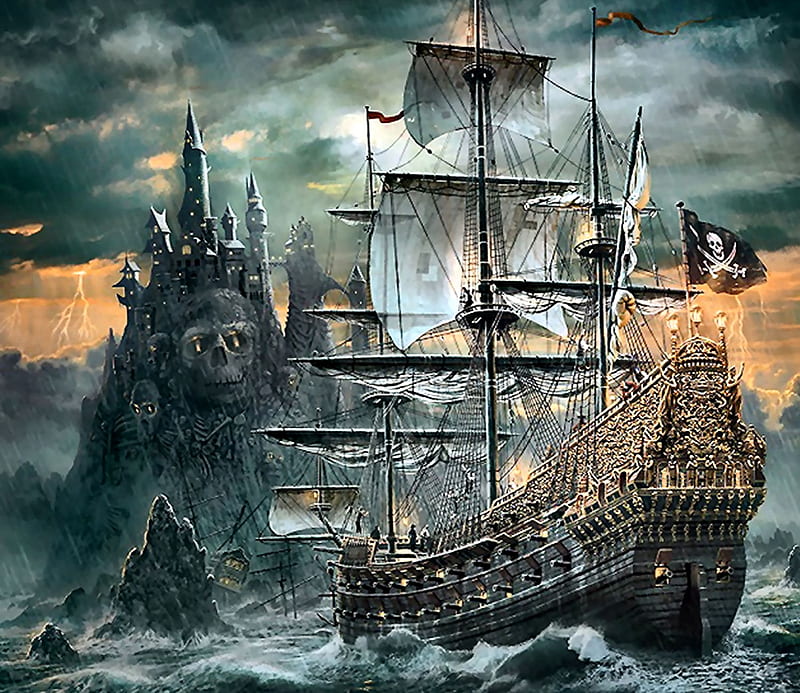In this captivating digital painting of a pirate ship, the scene captures an elaborate, old-style Spanish galleon from the 1600s, adorned with intricately carved golden details along its pitch-black wooden hull. The ship, decked with multiple white sails and a black pirate flag emblazoned with a skull and crossed swords, is brimming with activity, with various figures navigating the tumultuous seas. Glistening with the sporadic flashes of lightning, the dark, stormy sky casts an ominous yet thrilling glow over the entire setting. The pirate ship surges towards a foreboding coast dominated by a large black cliff, atop which stands a massive, blackened castle. This towering fortress is further enhanced by the eerie presence of a giant stone skull etched into the cliffside, surrounded by carved skeletons. The crashing waves and rain-soaked air amplify the treacherous, adventurous mood, making the entire scene steeped in mystery and fantasy.